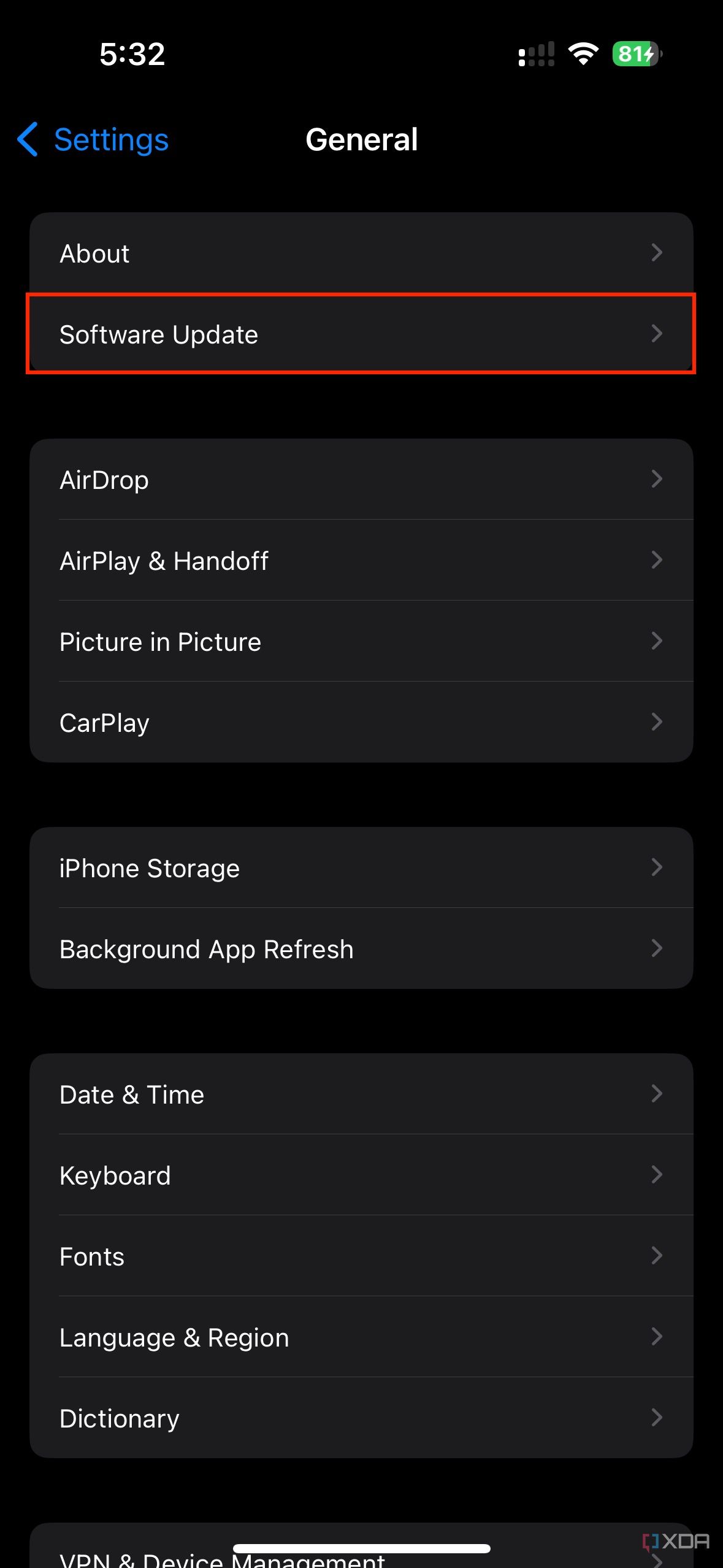The image depicts a general settings screen on an iPhone in dark mode. The interface appears vertical, suggesting it is more likely a phone rather than a tablet, though the possibility remains. The background is black with dark gray sections and white text, creating a sleek contrast. 

In the upper left corner, the white text displays the time as 5:32. The upper right corner shows the battery level at 81%, a full Wi-Fi signal, and a 1 out of 4 data coverage indicator. At the top of the screen, a blue back arrow is followed by the word "Settings" in blue, and the title "General" in white.

Below this header, the screen lists various clickable categories, starting with "About," followed by "Software Update" which is highlighted in red. Subsequent options include "AirDrop," "Airplane Handoff," "Picture-in-Picture," "CarPlay," "iPhone Storage," "Background App Refresh," "Date & Time," "Keyboard," "Fonts," "Language & Region," "Dictionary," "VPN," and "Device Management."

Notably, an XDA logo is positioned in the bottom right corner, confirming that the device is indeed an iPhone based on the available settings options.